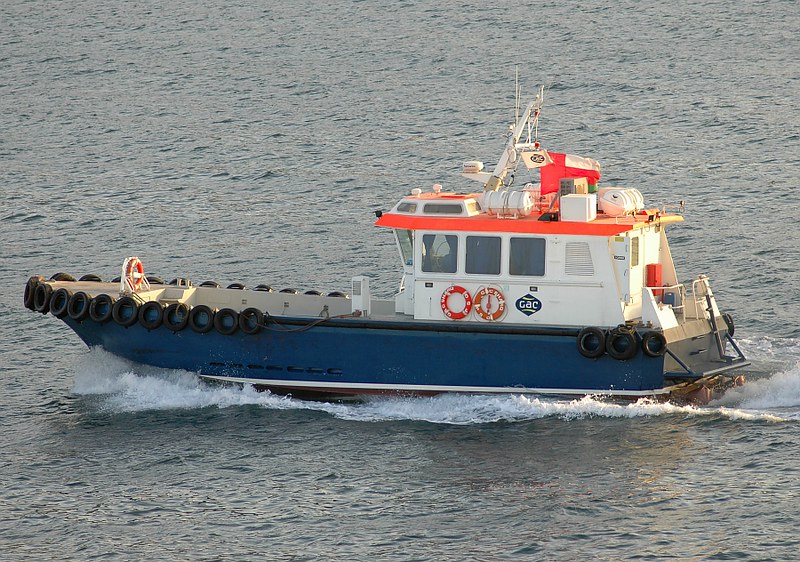Amidst the gray-blue expanse of the sea during the day, a distinctive ship, resembling a Coast Guard vessel, commands the center of the image. The water, predominantly gray with subtle hints of blue, sets a serene yet somber backdrop. The ship itself is designed for functionality and safety. Its hull is painted blue, while the cabin, occupying the aft section, is white with a trim of light red at the top. This cabin is enclosed, featuring several windows, and is equipped with multiple antennas on the roof, hinting at its role in communication and navigation.

Supporting its identity as a rescue ship, life rafts are visible on either side, and tires are strategically placed along the top edge of the blue-hulled section, likely for added protection and durability during rescue operations. The vessel is actively moving towards the left of the frame (the nine o'clock position), and this is evidenced by the dynamic wake billowing around it.